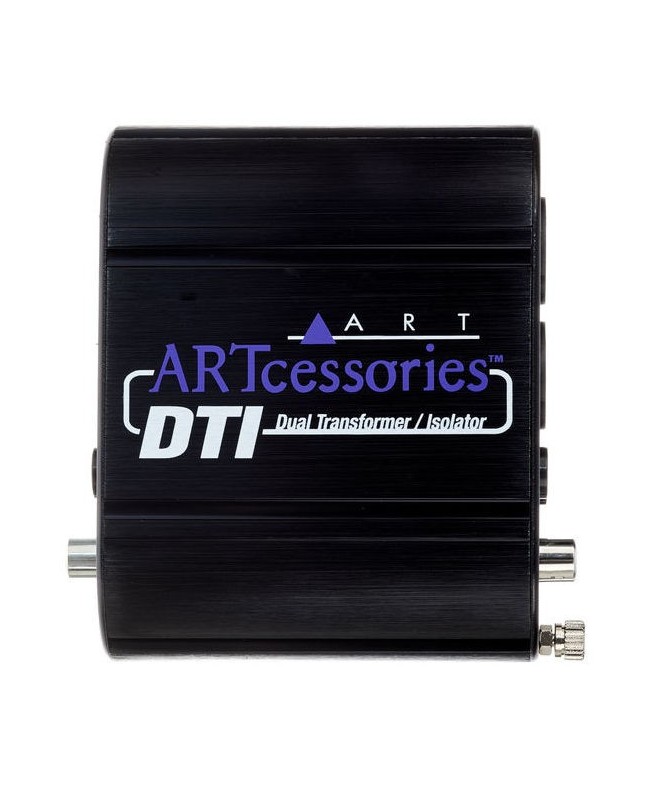This image depicts a black, rectangular, dual transformer/isolator device with various ports on its sides. The front of the device prominently features the text "ART" in white capital letters, which is underlined by a white line. To the left of the "A" in "ART" is a purple triangle. Below this, in purple text, appears the word "ARTcessories" with a trademark emblem. Further down, in white lettering, it states "DTI" and beneath that, in smaller font, "dual transformer / isolator." These texts are layered over a white rectangular outline that intersects some of the wording. The bottom section of the device has a large hand screw located on the bottom right corner, which appears to allow access to internal components. The device has more ports on the right side than on the left, although the exact number of ports is difficult to determine from the top-down view of the image.